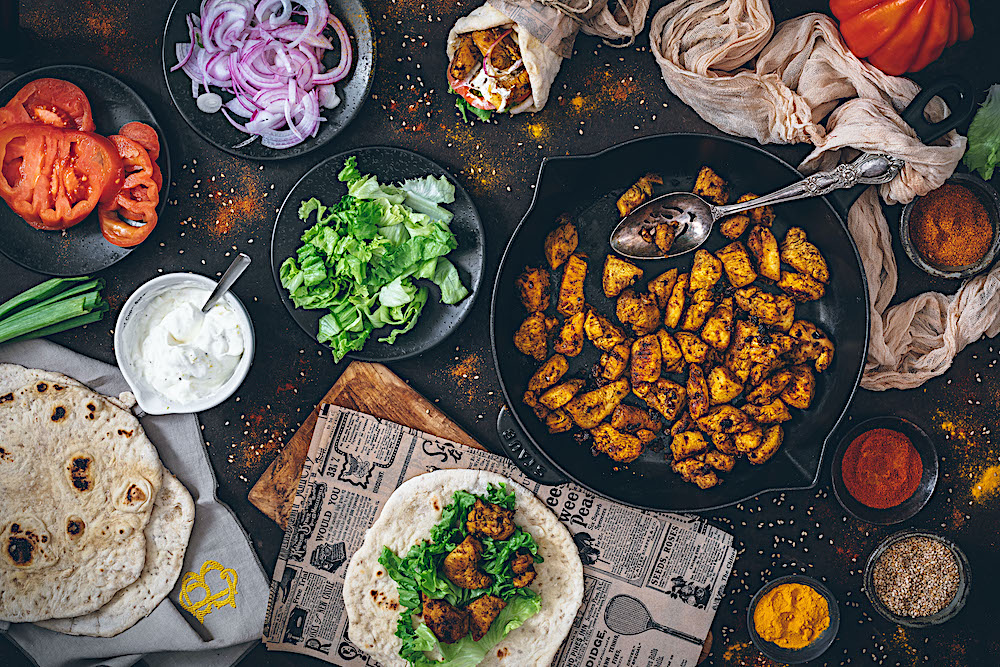The image depicts an enticing spread of Mexican-inspired cuisine laid out on a dark table. A black skillet, positioned just to the right, holds browned chicken accompanied by a large silver spoon. Surrounding the skillet are several small black containers; one contains salsa, another cheese, and a third possibly beans. In the upper left quadrant, a series of black plates feature an array of vibrant vegetables: sliced onions (both white and purple), shredded lettuce, and diced tomatoes. Just beneath these plates, resting on what appears to be a newspaper, a tortilla has been meticulously assembled with the browned chicken and crisp lettuce, ready for consumption. In addition, there's a white bowl of sour cream with a silver spoon nearby. Various tortillas, some plain and some already stuffed, are scattered on napkins throughout the setting. An orange pepper and some additional seasonings enhance the colorful presentation, suggesting a non-traditional, yet healthful Mexican meal. The overall scene is vibrant with hues of green, red, orange, and white, creating an inviting and appetizing visual feast.